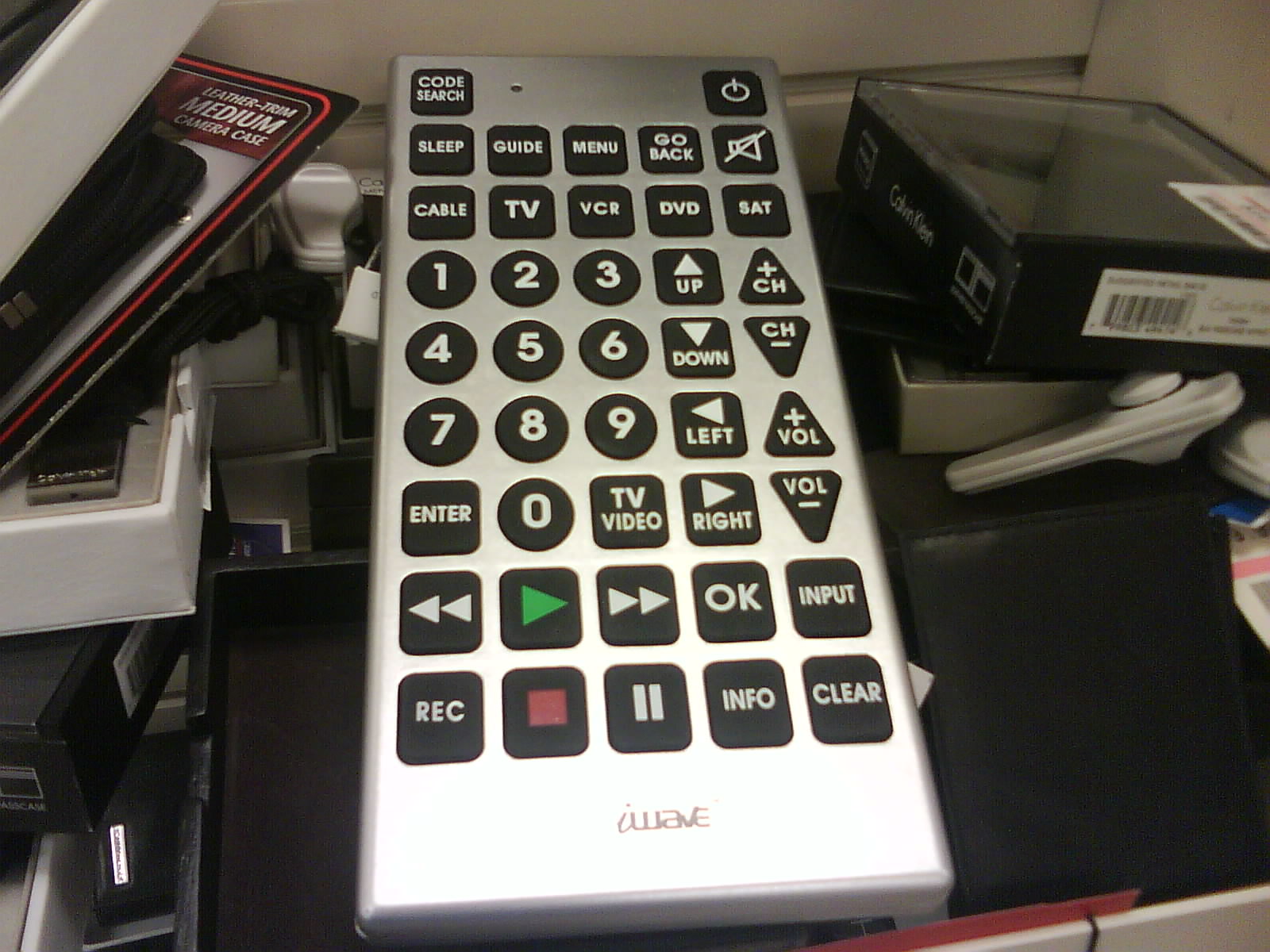The photograph features an old-fashioned, rectangular silver remote control labeled "iWave" at the bottom. This universal remote is designed for various audiovisual devices, as evidenced by the multitude of buttons: numerical pad (1-9, 0), enter, OK, REC (record), sleep, cable, TV, VCR, DVD, guide, menu, go back, satellite, play, pause, stop, rewind, fast forward, input, info, clear, volume up/down, and channel up/down. The remote control also includes directional arrows for navigation and additional functions like code search, mute, and an on/off button. The remote is situated amid a cluttered background of mixed items, including various boxes, security tags, shallow letter holders, and a packaging label indicating a "leather trim medium camera case," suggesting the area may be a disorganized storage space or junk drawer for tech-related items.